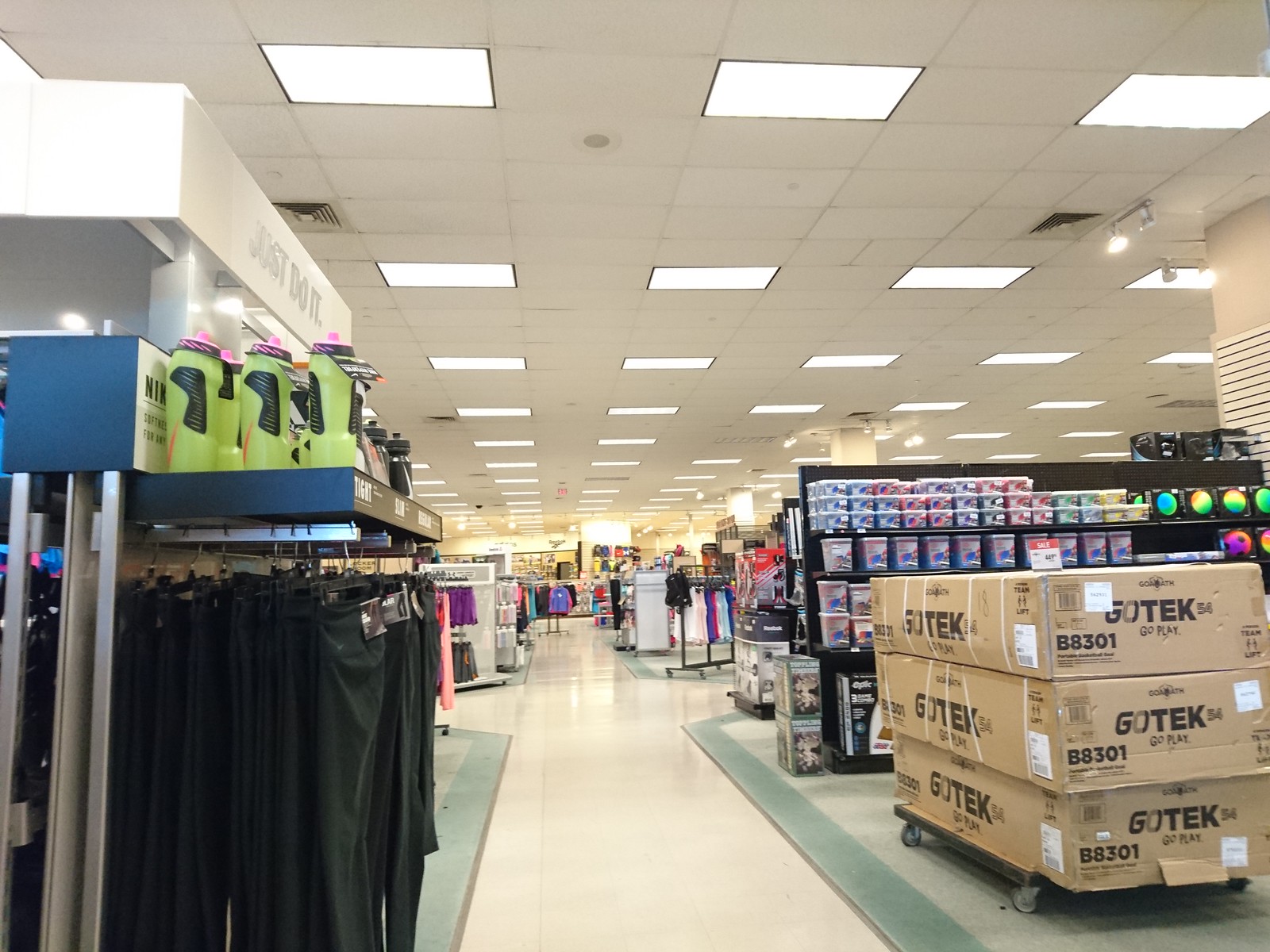This photograph captures the interior of a sporting goods store. The image is taken down an aisle, beginning at one end and extending towards the middle of the picture. On the left side, there's a rack adorned with black women's athletic stretch pants on hangers, positioned below green water bottles with black handles and purple tops. Above this display, a white shelf prominently features the Nike slogan "Just Do It" in light gray.

On the right side of the aisle, three large cardboard boxes labeled "Go Tech" are secured with plastic banding and placed on a wheeled dolly. Behind these boxes, a black shelving unit holds numerous plastic containers. Colorful multicolored balls, including a standout soccer ball with a rainbow gradient instead of the traditional white, are also visible on this side.

The flooring beneath is a tan color, flanked by areas of carpet. The store's drop ceiling, which includes white tiles and fixtures, houses fluorescent lights and speakers at regular intervals. In the distance, additional racks of athletic clothing can be seen, contributing to the store's dynamic and organized layout.